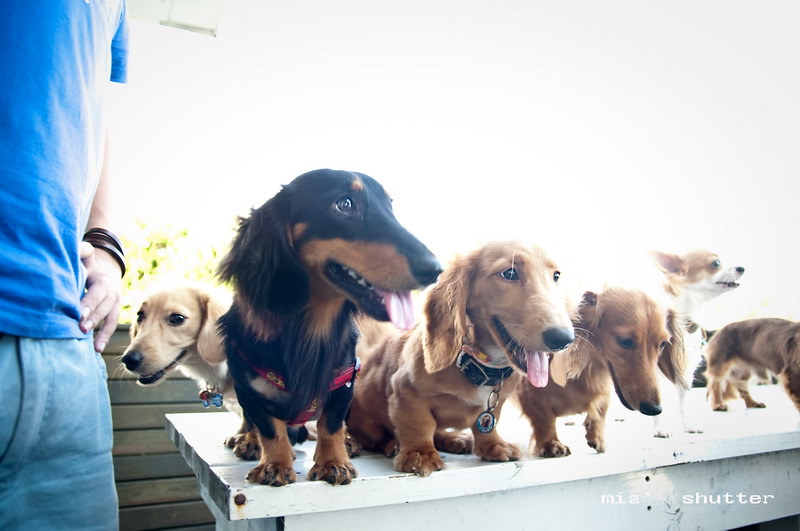The photograph captures a charming scene outdoors, dominated by a white wooden bench filled with six small dogs, mostly dachshunds, displaying a variety of coat colors including tan, black and brown, brown, and white with brown patches. The dogs are standing on the bench, some with their tongues out, appearing alert and engaged, possibly looking towards something to the left of the frame. The background is notably out of focus, featuring bright light and some indistinguishable vegetation, lending an airy feel to the image. To the left, partially in the frame, stands a fair-skinned individual dressed in blue jeans and a short-sleeve blue shirt, accessorized with dark bracelets on their wrist. The person's torso, hip, and a glimpse of their arm are visible, but their face is out of shot. The bottom right corner of the photograph bears the marking "MIA Shutter," suggesting the photographer's signature or watermark.